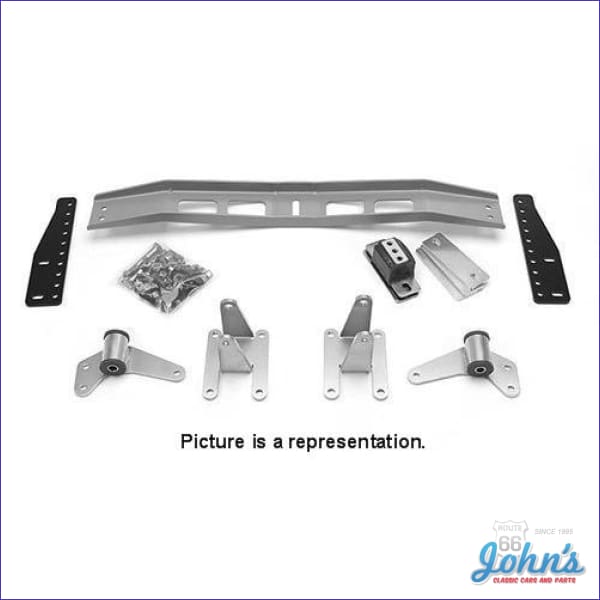The advertisement features a white background that dominates the scene, showcasing a variety of metallic parts meant for mounting a TV. Centrally positioned is a curved, silver metal piece with four large rectangular holes, two at each end, intended for screws. Flanking this central piece are smaller, flat black metal pieces, each adorned with numerous holes along their longest sides and a few on the opposite shorter sides. Scattered around are bags of screws, nuts, and bolts, indicating how the assembly is put together. At the bottom of the image, a message in black text states, "Picture is a representation." Additionally, the bottom right corner of the image features a light, faint gray Route 66 logo, with "John's" in blue script above the words "Classic Cars and Parts" in red text.